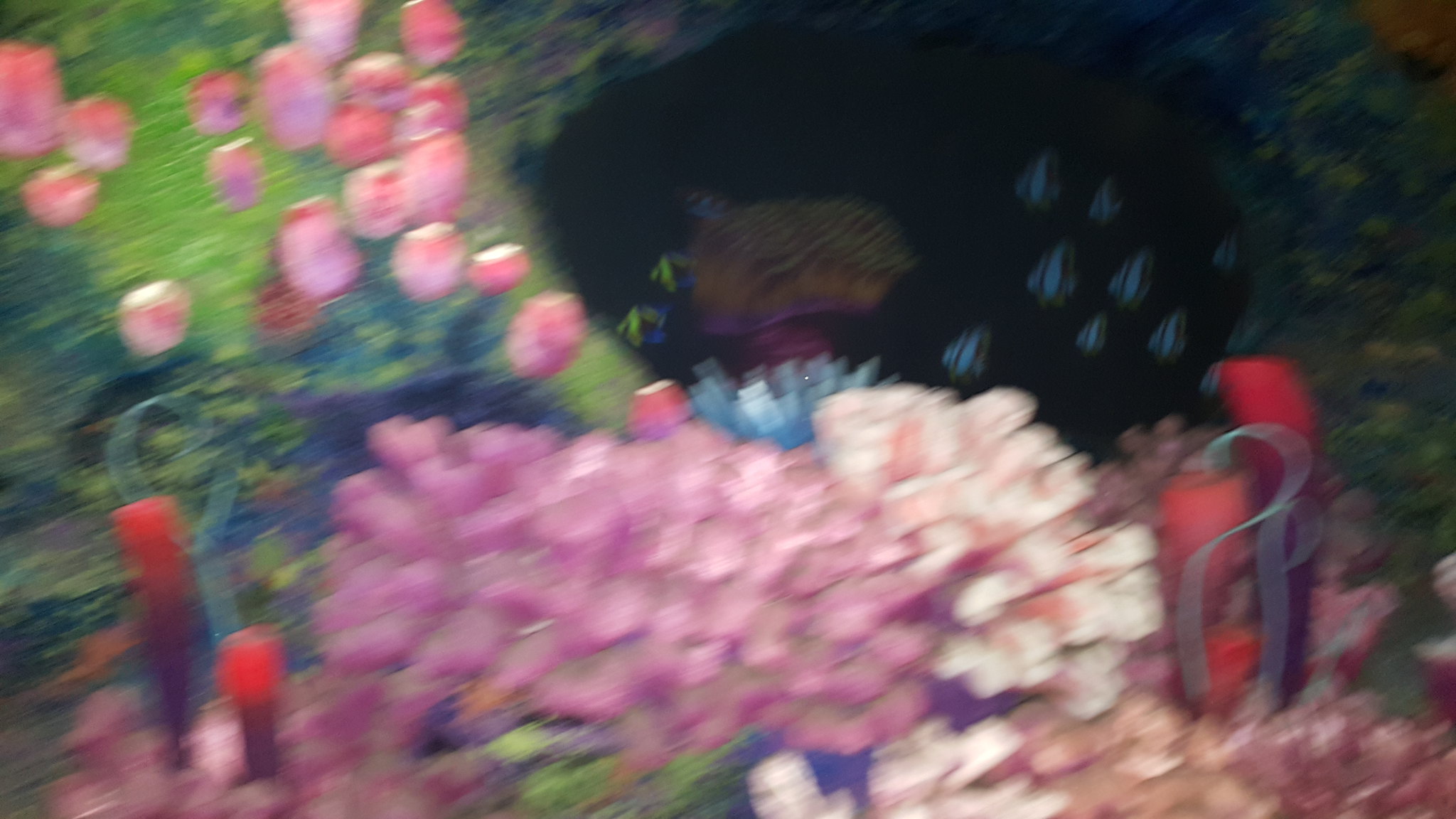In this rectangular image, we see a photograph characterized by a blurry yet vivid appearance, suggesting both a realistic and digitally altered quality. The lower half of the image features a softened vision of flowers, resembling roses, with light pink blooms on the right, light purple on the left, and additional light pink roses at the top, all set against a green background. In the lower right area, a red apparatus, possibly part of a garden installation, is spotted alongside what appears to be a sheer white scroll of fencing. The background, which has been digitally enhanced, depicts raindrops descending against a bright blue center with a translucent exterior, all set against a black backdrop.